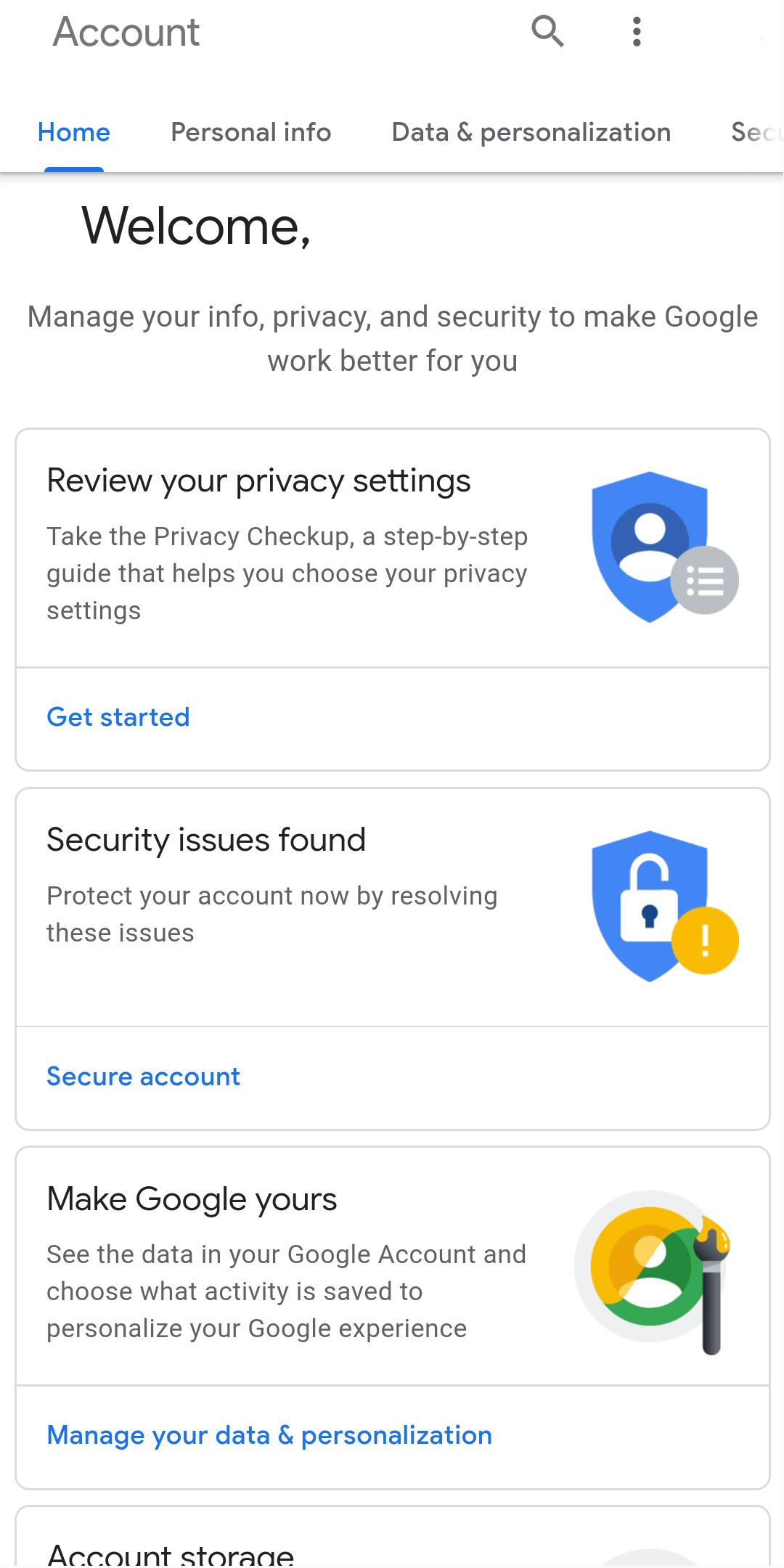This image displays the Google Account settings page. In the upper left corner, the word "Account" is prominently displayed. On the right side, there is a search icon and a vertical ellipsis menu (three dots stacked vertically).

Below the main header is a horizontal navigation strip with the options: "Home," "Personal Info," and "Data & Personalization." The "Home" tab is currently selected, highlighted in blue with a blue underline, while the other tabs are in gray. 

Following this, a gray line spans the width of the page. Just below, the text "Welcome" is displayed, followed by a prompt: "Manage your info, privacy, and security to make Google work better for you." The page highlights several actionable items, each with descriptive text and icons:

1. **Review your privacy settings**:
   - Icon: A shield with a person on it, next to a circle with bulleted lines.
   - Description: "Take the Privacy Checkup, a step-by-step guide that helps you choose your privacy settings."
   - Action Button: "Get started" in blue.

2. **Security issues found**:
   - Icon: A shield with an unlocked padlock, next to a circle with an exclamation mark.
   - Description: "Protect your account now by resolving these issues."
   - Action Button: "Secure account" in blue.

3. **Make Google yours**:
   - Description: "See the data in your Google Account and choose what activity is saved to personalize your Google experience."
   - Action Button: "Manage your data & personalization" in blue.

At the bottom of the visible section of the image, the text "Account storage" appears but the details are cut off. The layout organizes information efficiently with clear, distinctive icons and actionable steps to guide the user through managing their Google Account settings.